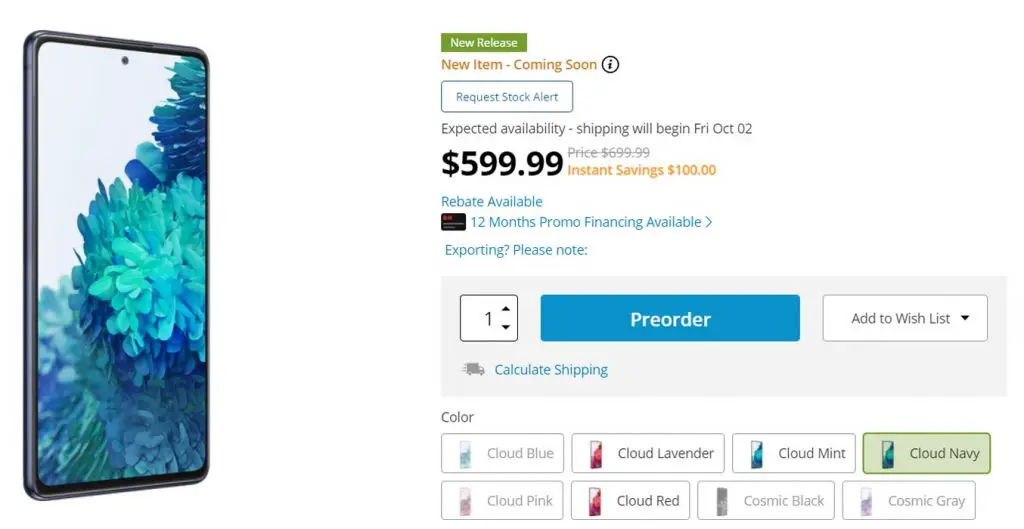**Detailed Image Caption for Web Page Advertisement:**

The web page features a promotional advertisement for a newly released cell phone. On the left side, there's a vibrant image of the cell phone with a colorful, abstract watercolor background, which resembles a mix of floral patterns and random color splashes. Centrally, within a green rectangle, bold white letters announce "New Release." Just below, a red label indicates "New Item Coming Soon."

In a structured layout: 
- A white square with blue text prompts users to "Request Stock Alert."
- Black text states the "Expected Availability" date.
- An indication that "Shipping will begin Friday, October 2nd" is provided.
- The bold black price is marked at $599.99, originally priced at $699.99, showcasing an instant saving of $100 in red.
- Information on "Rebate Availability" and "12 Months Promo Financing" is mentioned.
- A note on exporting is briefly highlighted.

Below, a large gray rectangle frames a white box outlined in gray, featuring a number "1" and accompanied by up/down arrow buttons to adjust the quantity. Below this section, a blue "Pre-order" button and an "Add to Wish List" button are accessible. Further down, an option to "Calculate Shipping" is available.

For color selection, the available options are presented in two rows of four rectangles each, listing the colors: Cloud Blue, Cloud Lavender, Cloud Mint, Cloud Navy, Cloud Pink, Cloud Red, Cosmic Black, and Cosmic Gray.